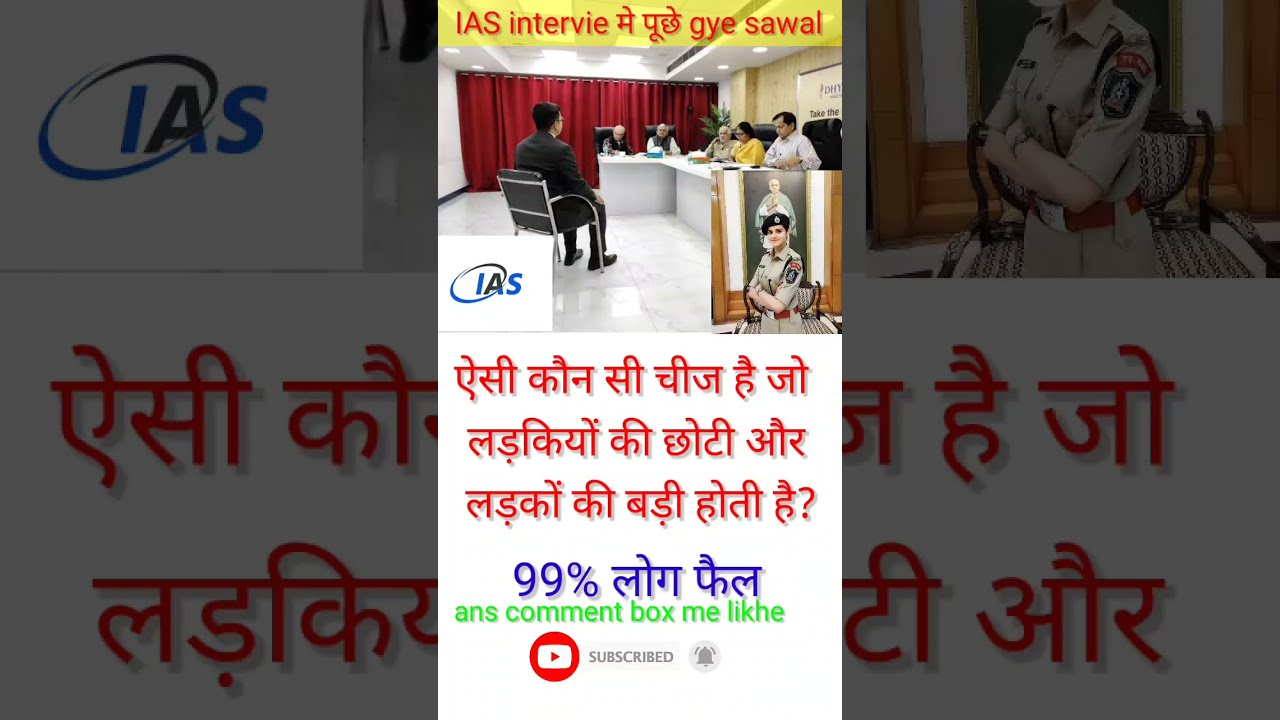The image depicts a formal interview setting, potentially related to a legal or political environment. At the top of the image, there is a white bar with unreadable red writing in a foreign script, likely Middle Eastern or Indian. The background features a white room with a wooden motif on the right side and closed red curtains along the back wall. Seated at a table are five people, including four men and one woman, the latter wearing a bright yellow outfit. In front of them sits a bespectacled gentleman in a black suit, possibly the interviewee, facing the panel. There is another image within the main image showing a woman in a military or police uniform with her arms crossed. Below the images, there are three red text bars, followed by numbers in blue reading 99%, and more text. Green lighting displays the phrase "ANS comment box me, L-I-K-H-E," accompanied by a YouTube logo, a "subscribe" prompt, and a gray notification bell icon. The scene and accompanying text suggest this might be an advertisement for a social media video or a recorded interview.